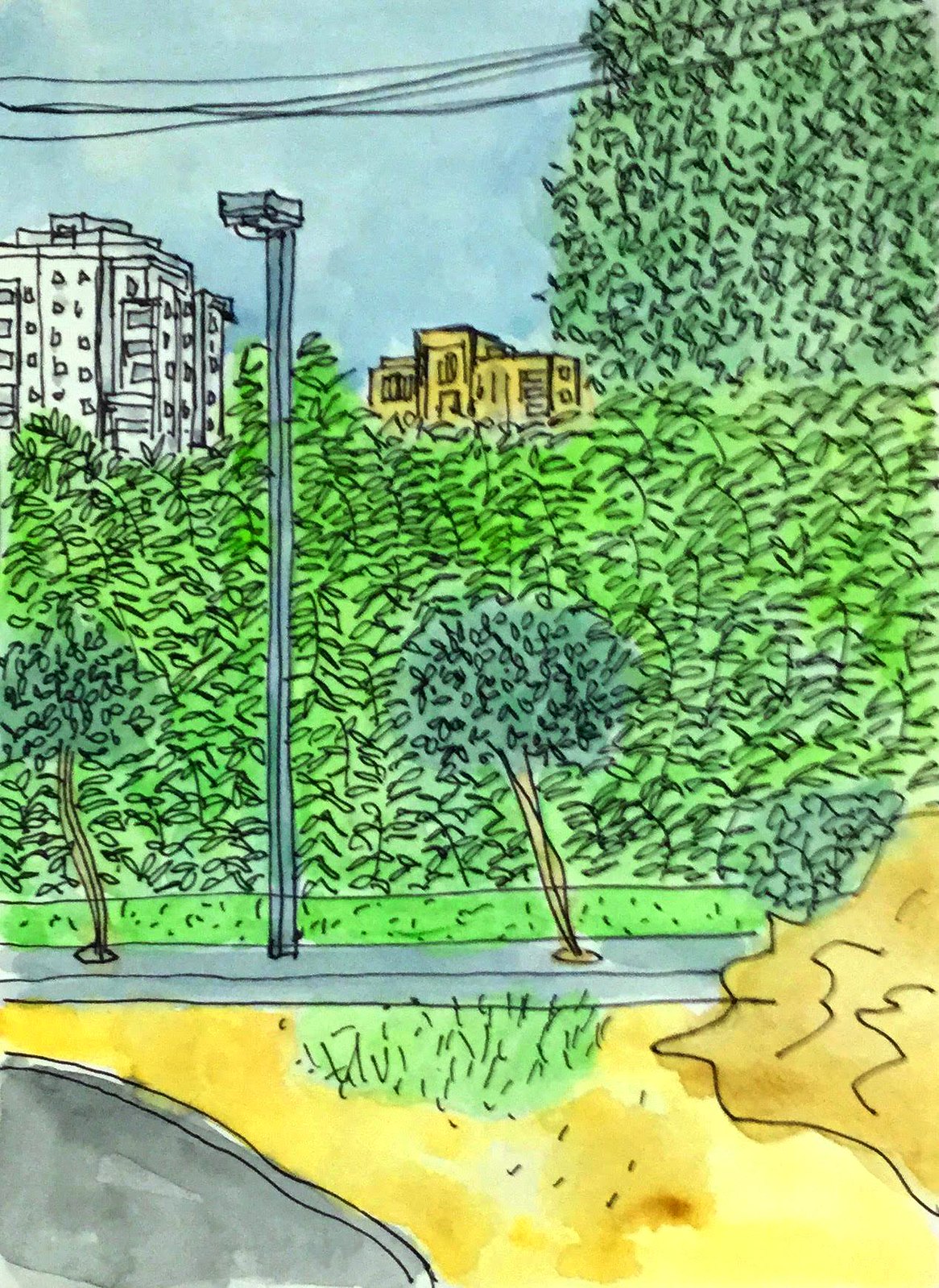This artwork depicts a serene park scene within a vertically elongated, rectangular frame. The background is graced by a clear blue sky, lightly punctuated by glimpses of buildings peeking through the lush foliage. Among these, a multi-story white building stands on the left, while a yellow building is partially visible towards the top center, both artfully obscured by the greenery. To the right, a prominent, large green tree anchors the composition.

Foregrounding the scene is a dense, sketchy row of green bushes, delineating the buildings from the park area. In front of this verdant barrier is a curb or sidewalk, evident by a sketched streetlight and a trio of smaller trees or possibly two small trees and a hedge to the right.

Closer to the viewer, the ground appears sandy with patches of sparse grass, suggesting a well-trodden path or playground area. The bottom left corner of the scene hints at a small body of grayish water, adding a cool, reflective element to the painting's warm, organic tones.